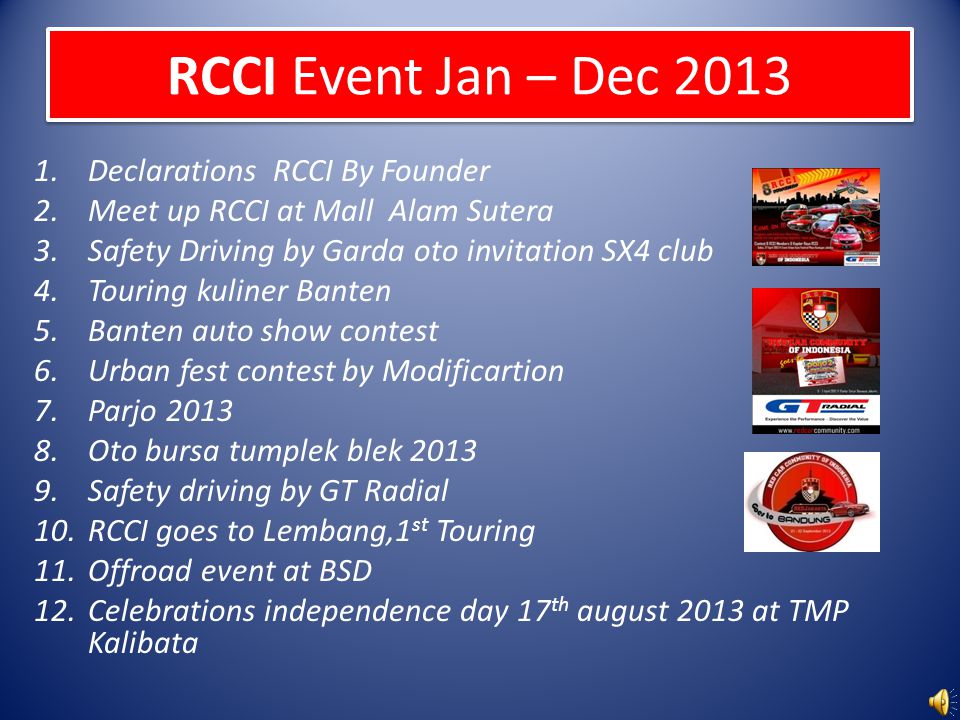This image is a detailed poster or slide announcing the RCCI event schedule from January to December 2013. The title, "RCCI Event January to December 2013," is prominently displayed in a red rectangular box at the top. The poster details 12 monthly events starting with the "Declaration of RCCI by Founder" in January and including activities such as "Meetup RCCI at Mall Alam Sutera" in February, "Safety Driving by Garda Auto Invitation SX Force Club" in March, and "Celebrations Independence Day" on August 17, 2013, at TMP Calibata. Additional events listed feature auto-related activities like touring, contests, and off-road events. The background is primarily blue with a vertical grid of three images on the right showcasing car races and promotional content. The poster's overall color scheme includes blue, light blue, white, red, black, yellow, and orange, giving it a vibrant and dynamic appearance, typical of a PowerPoint presentation.